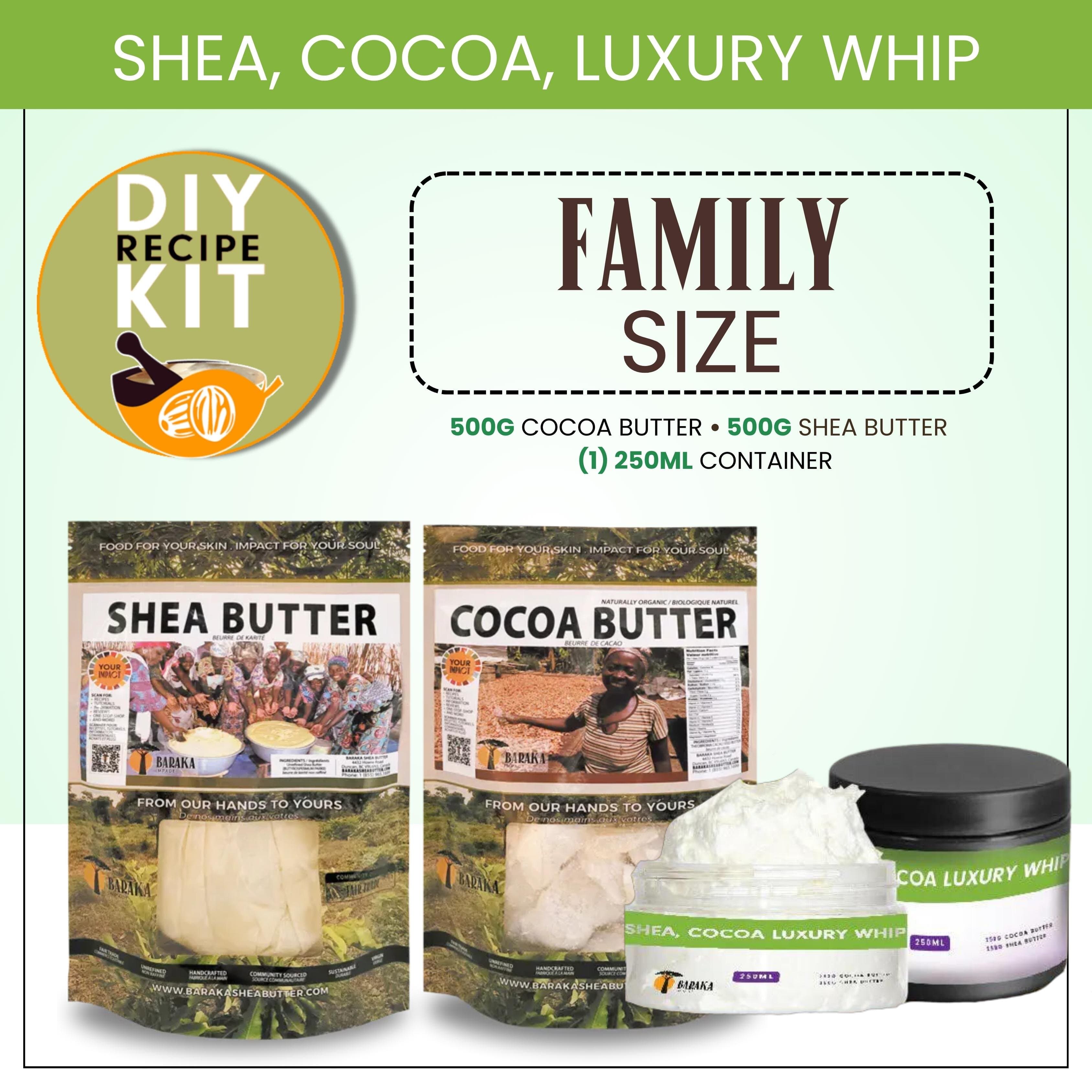The advertisement for Shea Cocoa Luxury Whip features a distinctive dark green header with white lettering, proclaiming the product name, "Shea Cocoa Luxury Whip." Below, the background transitions to a lighter mint green. On the top left, a circular badge outlined in orange reads "DIY Recipe Kit" in white lettering. Below this, an orange bowl with black-handled pestle is depicted, showing the mixing of ingredients. Adjacent to this, a black dotted border encloses the phrase "Family Size" in bold, black font. 

Detailed ingredients follow beneath, denoting "500 grams of cocoa butter" and "500 grams of shea butter" in brackets, alongside "one 250-milliliter container," rendered in dark green text. The center presents two product bags: the left bag is for shea butter, featuring an image of women in traditional dress making shea butter in large vats against a greenish backdrop. The tagline "From Our Hands to Yours" is prominently displayed. The right bag is for cocoa butter, showcasing a woman pointing towards an area of production, adorned with the same tagline and an African tree motif.

To the right of these bags, two jars of Shea Cocoa Luxury Whip are displayed. One jar is open, revealing the white, fluffy whip reminiscent of whipped cream. The other jar remains sealed, featuring a white lining at the bottom and a green banner with white lettering encircling the jar, capped with black. The banner reads "Shea Cocoa Luxury Whip," epitomizing the luxurious and handmade qualities of the product.